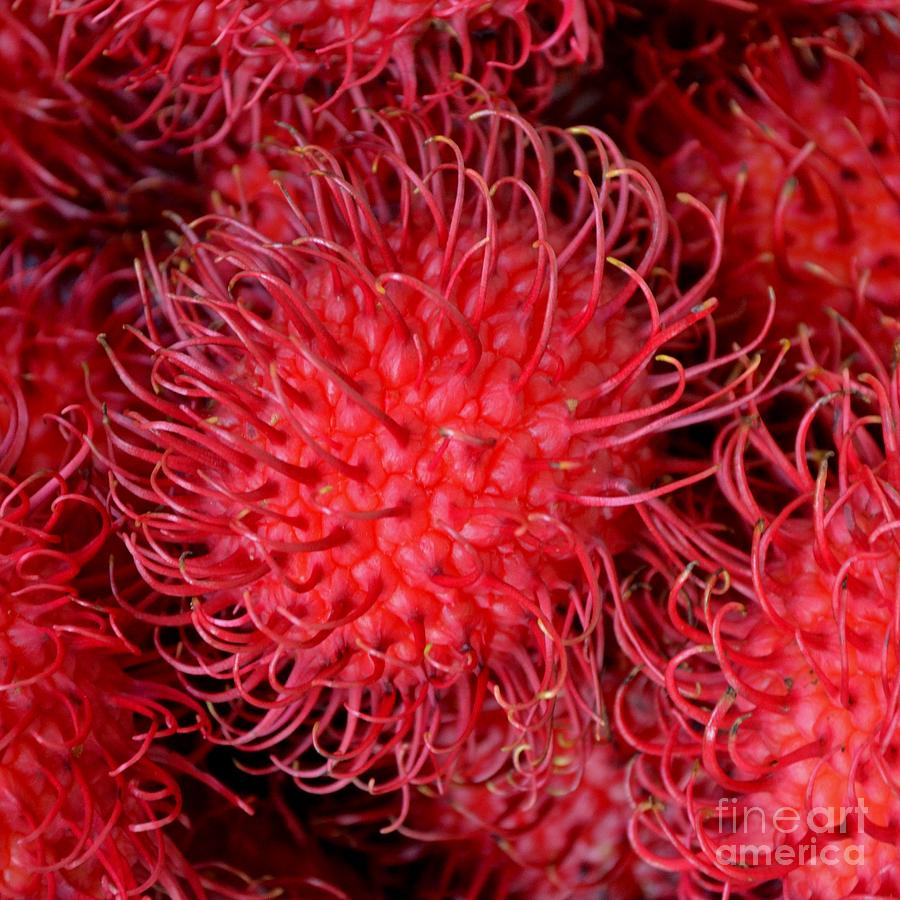The image is a detailed, close-up view of roundish, red or dark pink objects that bear a striking resemblance to coral or sea sponges, though they could also be a type of exotic produce. Each object features numerous small nodules across its surface, from which fine, crimson hair-like follicles emerge. These follicles often curl at the ends, showcasing green or lime-green tips with occasional hints of white or yellow. The composition shows a main central object surrounded by partial views of similar objects around the edges, creating a clustered, almost underwater scene. In the bottom right corner, faint writing reads "Fine Art America," suggesting the image is either an artistic photograph or painting. The backdrop is a contrasting dark black, enhancing the vivid colors and intricate details of these intriguing structures.